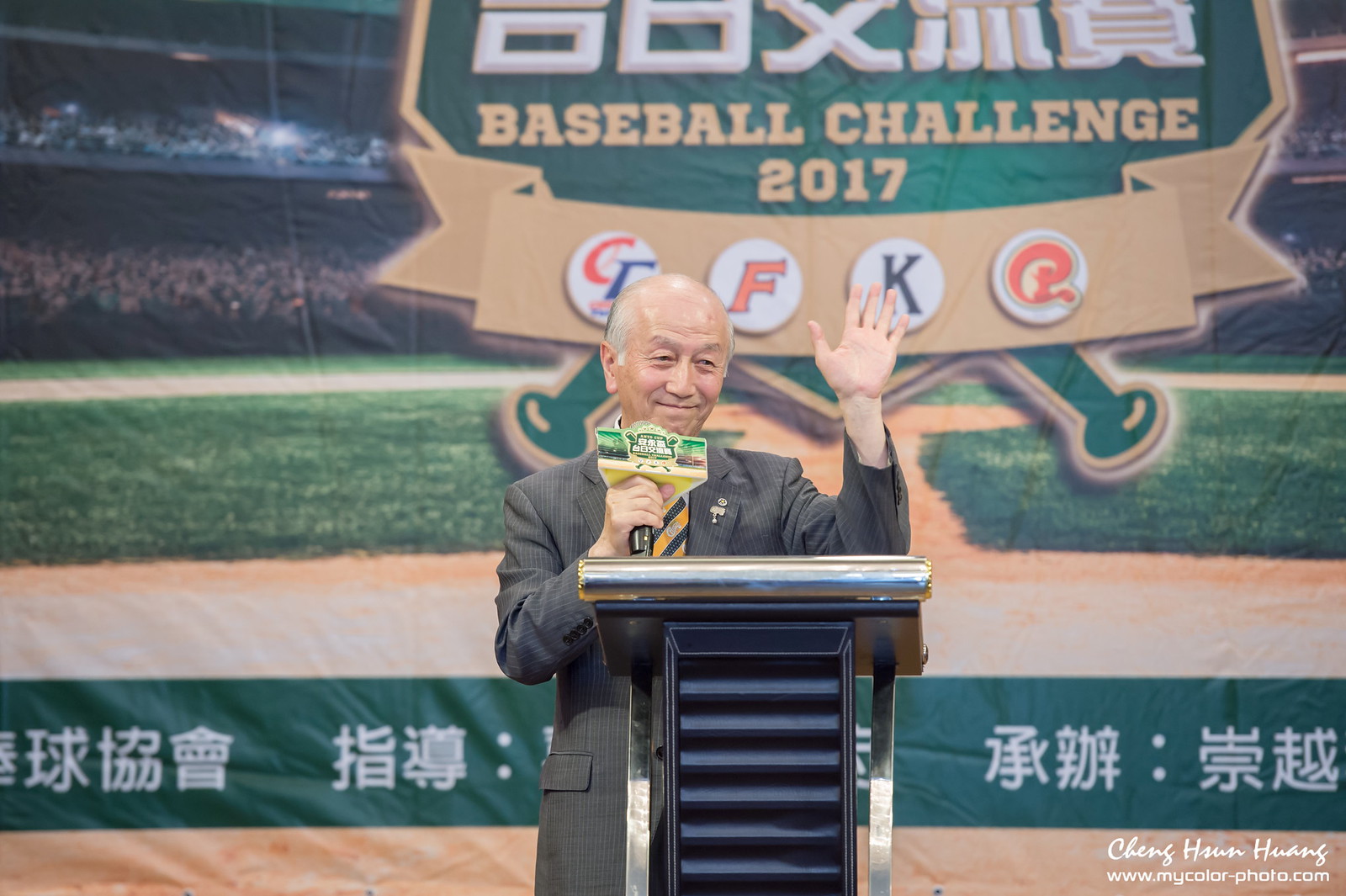The image portrays an older Asian gentleman, presumably from Taiwan or China, standing behind a podium adorned with blue and black stripes and a metal top. He is waving to the crowd while holding a microphone that sports a colorful top and a piece of paper with Chinese writing around it. The man is bald on top with gray hair on the sides and is dressed in a gray suit with a tie. Behind him, a large banner displays an image of a baseball field with a visible pitcher's mound, grass, and dirt paths, alluding to a significant crowd in attendance. The banner prominently features the text "Baseball Challenge 2017" with two crossed baseball bats and additional Asian characters. Four circles with different symbols, including an orange "C" and "F," a blue "T," a black "K," and an orange symbol resembling a "P," are visible. In the bottom right-hand corner of the image, white text credits the photographer, Cheng Hun Huang, and provides the website www.mycolor-photo.com.